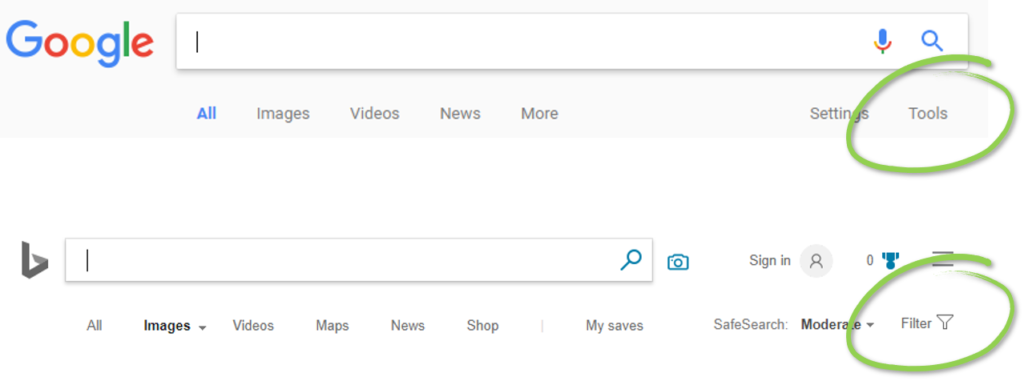The image depicts a screenshot of the Google search interface with a themed design. At the top of the page, there is a light blue box displaying the Google logo in its iconic blue, red, yellow, and green colors. Below the logo, there is a large search bar featuring a microphone icon on the left and a magnifying glass on the right. The word "All" is highlighted in blue beneath the search box, with options for "Images," "Videos," "News," and "More" listed in sequence.

Further down, the interface shows a green circled area around the "Tools" option, indicating it is emphasized or selected. A thick blue and black line starts at this point, vertically extending downwards and wrapping around a second search box, which mirrors the first one with its black line border and magnifying glass icon.

Adjacent to this area, a blue camera icon is prominent, symbolizing image search functionality. Additionally, there are buttons for signing in, a telephone icon, and a three-line menu icon representing more options or settings. Below these elements, a navigation bar lists various categories including "All," "Images," "Videos," "Maps," "News," "Shop," "My Sales," and "Safe Search," with "Moderate" and a filter option. The word "Filter" is also encircled in green, suggesting it is an active selection.